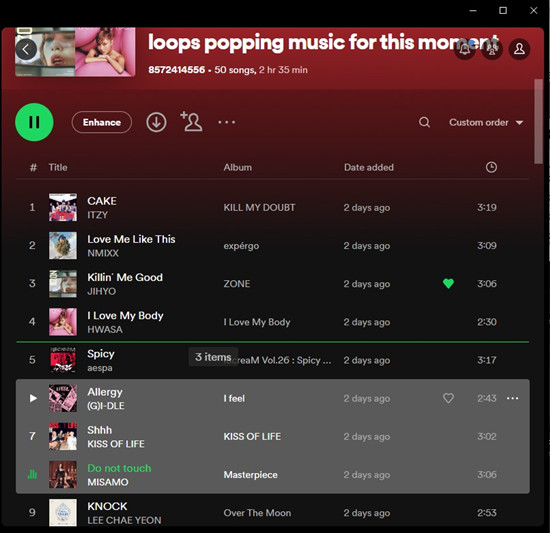This image is a screenshot of a Spotify interface, featuring a predominantly black background. At the top of the screenshot, there is a horizontal bar in a deep red or maroon color, which gradually fades into the black. Within this red bar, on the left side, there is a back arrow icon adjacent to two small album covers. To the right of these icons, in white text, it reads "Loops Popping Music For This Moment." Below this title, a smaller text indicates "50 songs, 2 hours 35 minutes."

Beneath this header, there are several interactive elements. A green circle with a black pause button is centrally located, and next to it is an "Enhance" button. To the far right, there's a series of icons: a down-arrow inside a circle, a person-add symbol, and then three vertically aligned dots for additional options.

Further down, against the dark background, there are column headers labeled with a hashtag (#), "Title," "Album," "Date Added," and "Time." A scroll bar appears on the right-hand side of the screenshot for navigation. Under each number, corresponding to the song's position in the playlist, there are details about the song, including the album thumbnail, album name, the date it was added, and the song’s total play time.

Notably, a green line is visible between the fourth and fifth numbers in the list, and the songs corresponding to numbers 6, 7, and 8 are highlighted with a grey block. It appears that the song at position number 8 is currently playing.